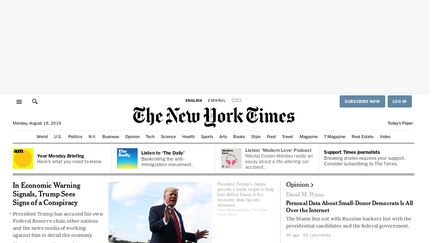This detailed caption describes an image that is a screenshot from the New York Times front page:

"The image captures the top quarter of the digital front page of the New York Times. Set against a white background, the screenshot prominently features the New York Times logo in large black font at the center top. To the left of the logo, near the top-left corner, a small magnifying glass icon represents the search function. Adjacent to this, on the upper right corner, is a blurry dark greenish-blue section with white text where 'Subscribe Now' appears on the left while a smaller 'Log In' button sits on the right.

Across the top, the language options 'English' and 'Español' are visibly displayed in black lettering. Below the logo, a horizontal menu bar with categories in black text runs from left to right, dividing the page content. Beneath this menu, a thick gray line separates the main content area.

The main content area begins with four short sections, each with brief descriptions: 'Your Monday Briefing,' followed by 'Listen to the' (with the last word obscured), 'Law Podcast,' and 'Support Your Journalist.' Icons accompany the first three sections on the left side.

Under another gray line, the headline 'In Economic Morning Signals, Trump Sees Signs of a Conspiracy' appears on the upper left. To the right of the headline is an image of President Trump with his upper body against a sky background, hands raised. On the far right, the 'Opinion' section headline reads 'Personal Data About Small Donor Democrats All Over the Internet' in bold black text. The date in the upper left corner is slightly blurred, indicating either 'Monday, August 18th or 19th, 2019.' The overall layout corroborates the authentic appearance of the New York Times’ digital front page."